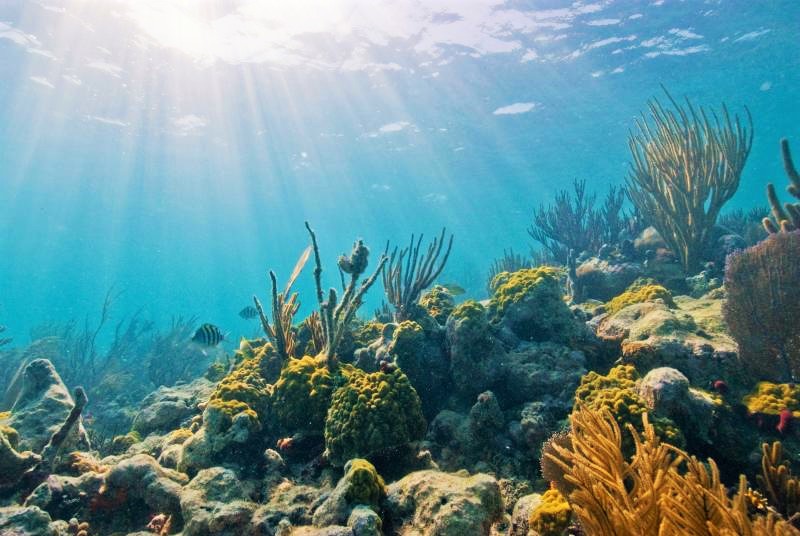This stunning underwater image captures a breathtaking scene beneath the ocean's surface. The water is a deep, vibrant blue with rays of sunlight piercing through from above, casting a magical glow on the scene. The seafloor is adorned with a variety of sea life, including diverse coral formations and rocks covered in green and brown vegetation and moss. Notably, an orange sea organism stands out on the bottom right corner, while long plants sway gently in the water. Amidst the coral and plant life, vibrant yellow fish with distinctive black stripes swim gracefully, enhancing the scene's surreal beauty. The image is so perfect and picturesque that it almost appears to be AI-generated.